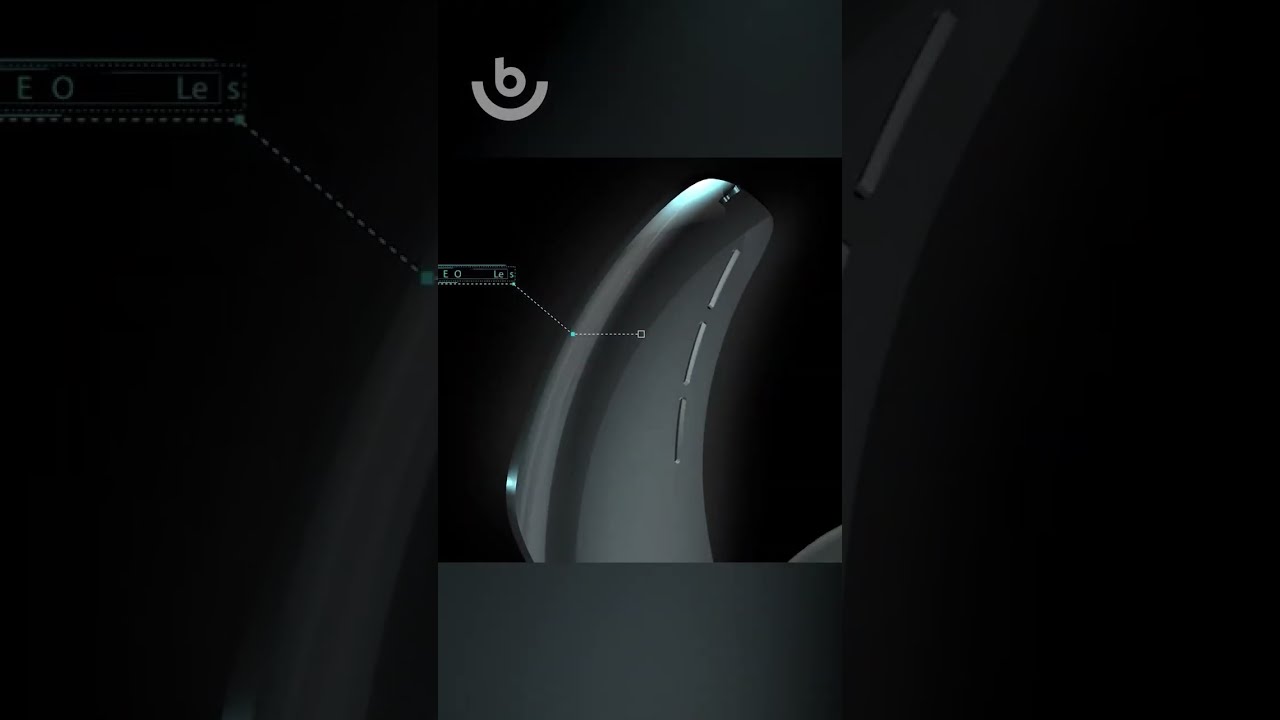This grayscale image features a central object with a complex, possibly metallic form, resembling part of a motorcycle saddleback or a curved pipe. The central object is broad at the bottom and narrows toward the top, exhibiting both light and dark gray sections. A dotted line extends from this object to a boxed area labeled with the letters "E-O-L-E-S." This label appears more prominently in an enlarged view on the left-hand side of the image. The right side displays an expanded view of three very thin, light gray vertical stripes. Surrounding the central image, the background is a zoomed-in version of the same object, creating a mirrored effect on the left and right sides. At the top of the image, there's a gray header with a lighter gray bowl-shaped stripe beneath a lowercase letter "b," resembling a smile. A similar gray footer resides at the bottom of the image. Overall, the dark composition and intricate details make the exact nature of the object challenging to identify.